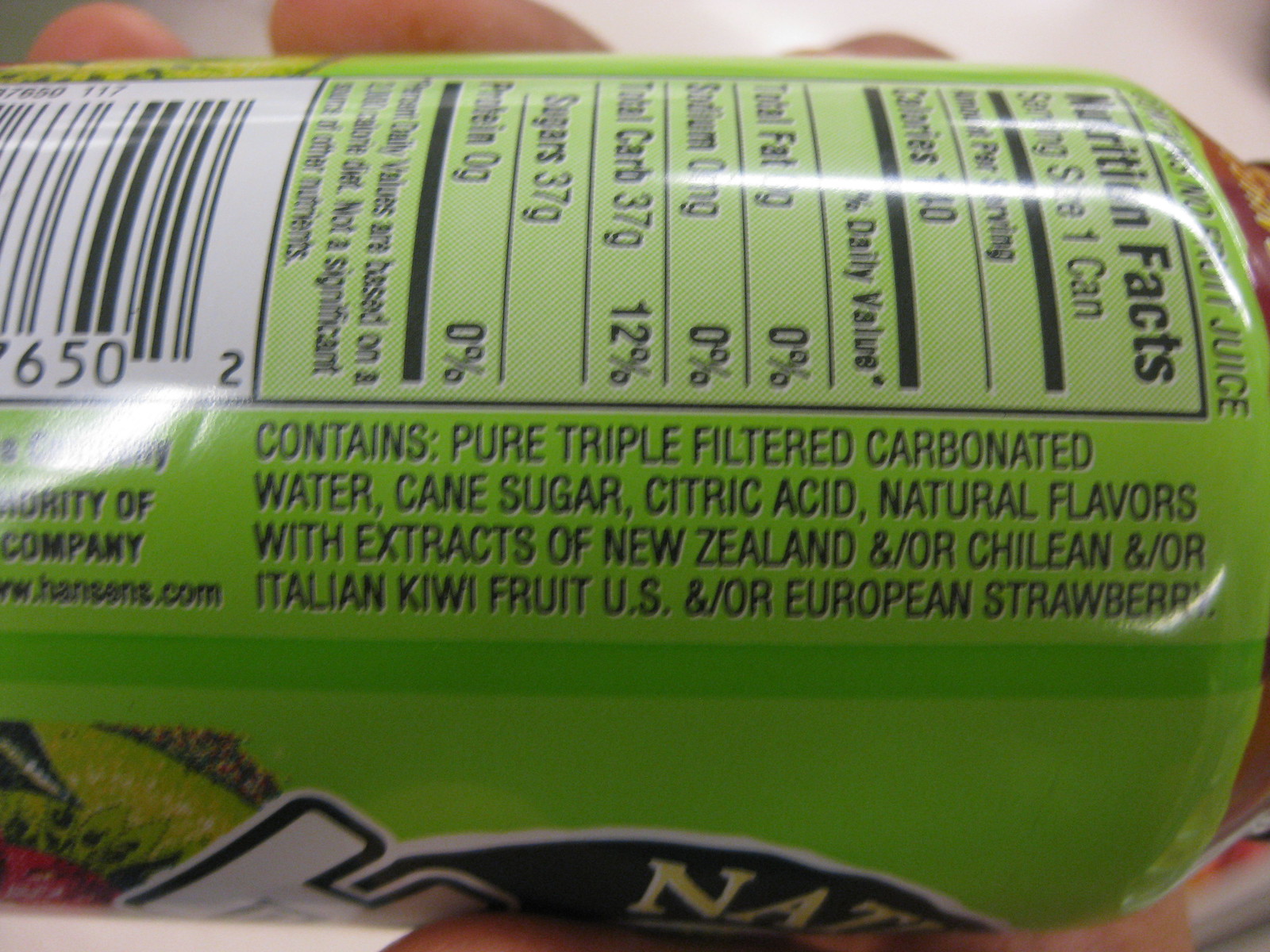This is a detailed side view photograph of a hand holding a can of juice drink. The fingers and fingertips are visible, firmly grasping the can. The central focal point of the image is the list of ingredients on the can, which prominently includes triple-filtered carbonated water, cane sugar, citric acid, natural flavors, and extracts of kiwi fruit (sourced from New Zealand, Chile, or Italy) and strawberries (sourced from the U.S. or Europe). Above the ingredients list, the nutrition facts are partially visible, noting that the serving size is one can. However, there's a glare from the light reflecting off the can, obscuring some details, making it difficult to clearly see the exact calorie count, which appears to be approximately 140 calories.